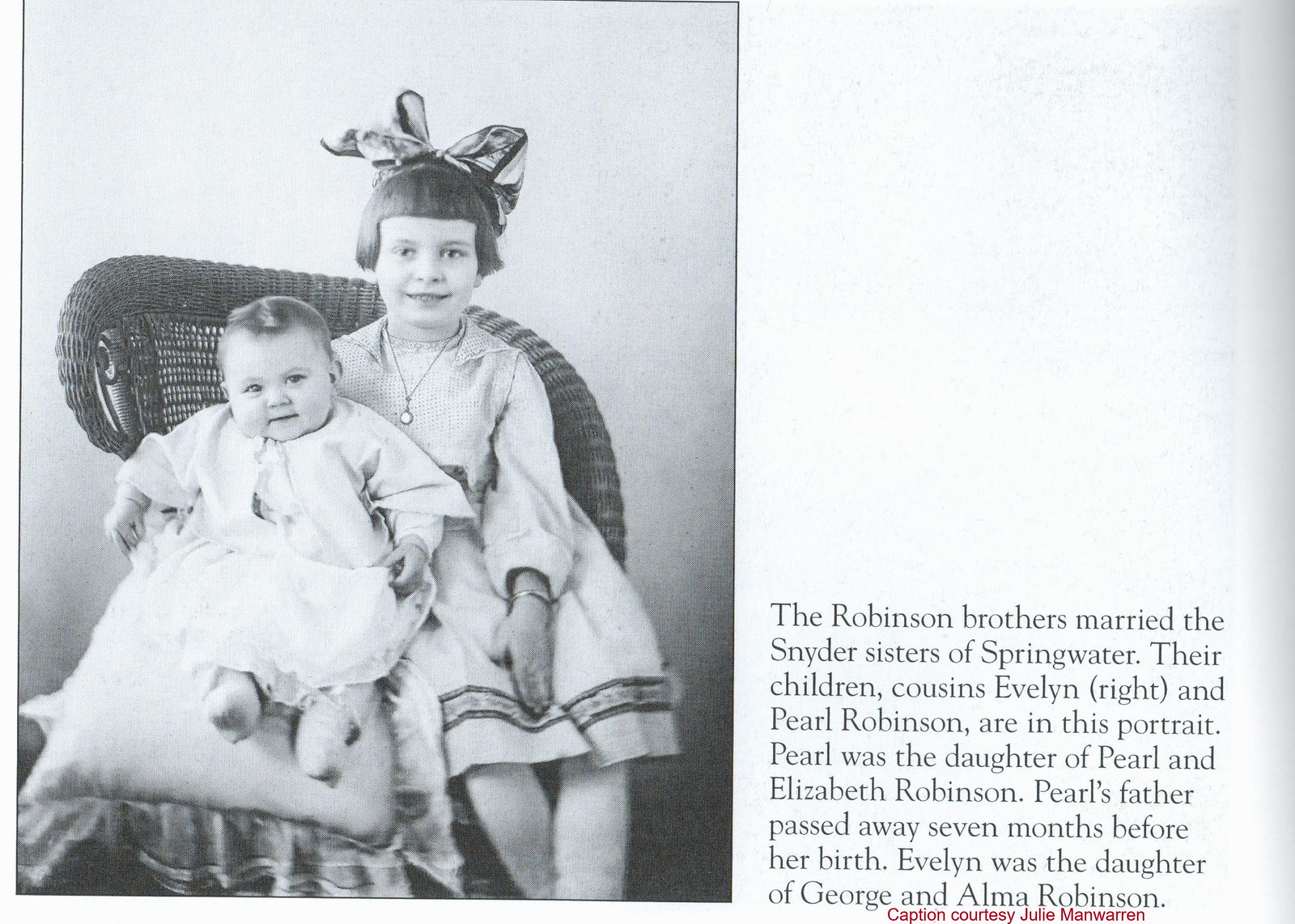This detailed black-and-white photo features two young children, Evelyn Wright and Pearl Robinson, seated in a wicker chair. Evelyn, likely around four or five years old, has a short haircut with bangs cut straight across her forehead and is adorned with a large bow in her hair. She wears a dress and a necklace, and lovingly has her arm around baby Pearl, who is dressed in a white gown and sits on a pillow. The right half of the image contains text describing the familial relationships: "The Robinson brothers married the Snyder sisters of Springwater. Their children, cousins Evelyn Wright and Pearl Robinson, are in the portrait. Pearl was the daughter of Pearl and Elizabeth Robinson. Pearl's father passed away seven months before her birth. Evelyn was the daughter of George and Alma Robinson." Below this text in red is the caption "Courtesy Julie Mann Warren."